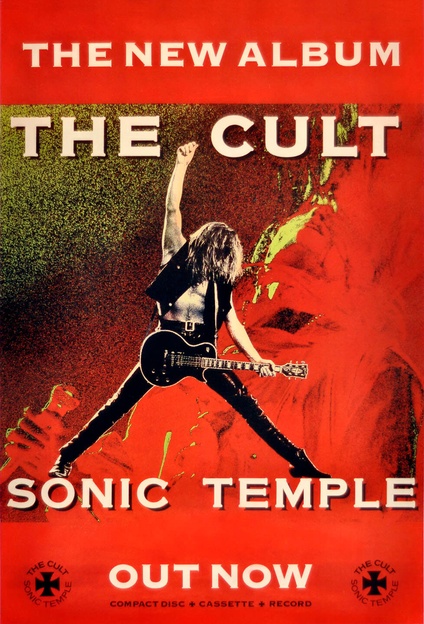The album cover features a predominant red background with sections tinged in green and black speckles. At the center, a bare-chested musician stands dramatically with his legs spread wide, clad in black leather pants, a black vest, and black shoes. His long, dark hair partially obscures his face as he holds a black guitar with his left hand, while his right arm is extended powerfully upwards. At the very top of the cover are the words "The New Album" in white capital letters, followed just below by "The Cult". Directly beneath the musician’s feet, in white capital letters, it reads "Sonic Temple". At the bottom of the cover, "Out Now" is prominently displayed in white, with "Compact Disc", "Cassette", and "Record" listed beneath in smaller black type. On both the bottom left and right corners, the emblem showcases the band's name and the album title, "The Cult - Sonic Temple". Additionally, in the backdrop, a subtle silhouette of another guitarist’s hand and headstock adds depth to the scene.